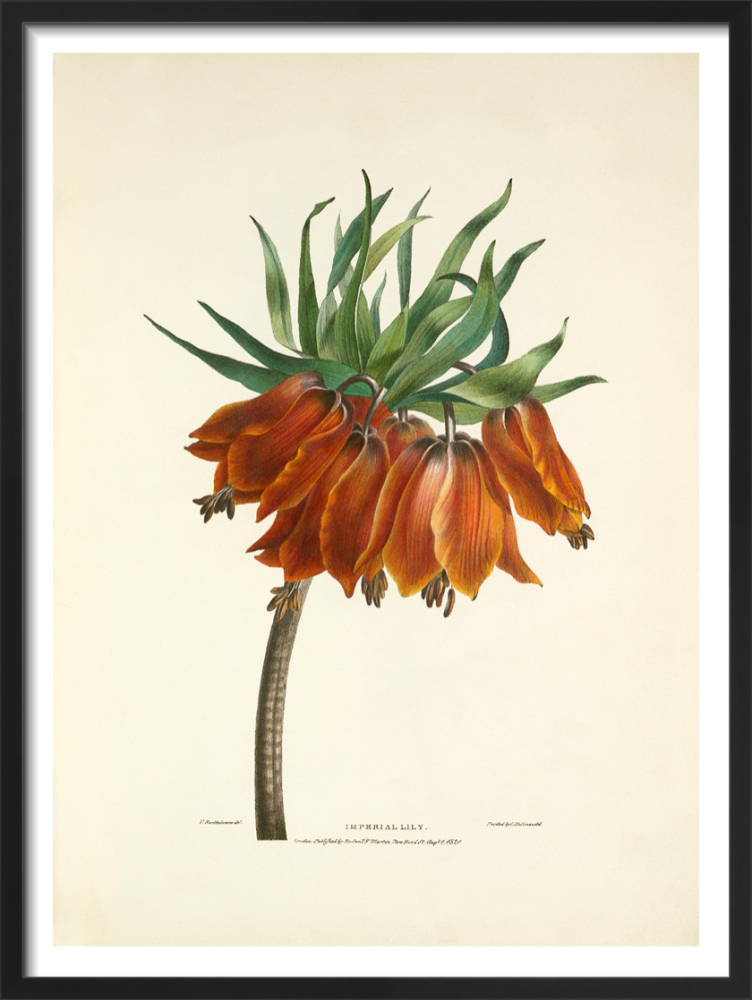This image is a detailed painting of an "Imperial Lily" encased in a black frame with a white inner border. Set against an off-white, manila background, the focal point of the artwork is a flowering plant characterized by a brownish stem that ascends upwards. The plant features four prominent flowers with ombre petals shifting from brown at the base to orange and hints of yellow towards the edges. The flowers hang upside down, displaying small antenna-like structures in the center, each tipped with pollen and surrounded by five or six tiny stubs. Reaching upwards, thin and stringy green leaves densely cluster at the top. Below the botanical depiction, the label "Imperial Lily" is visible with additional, unreadable text.